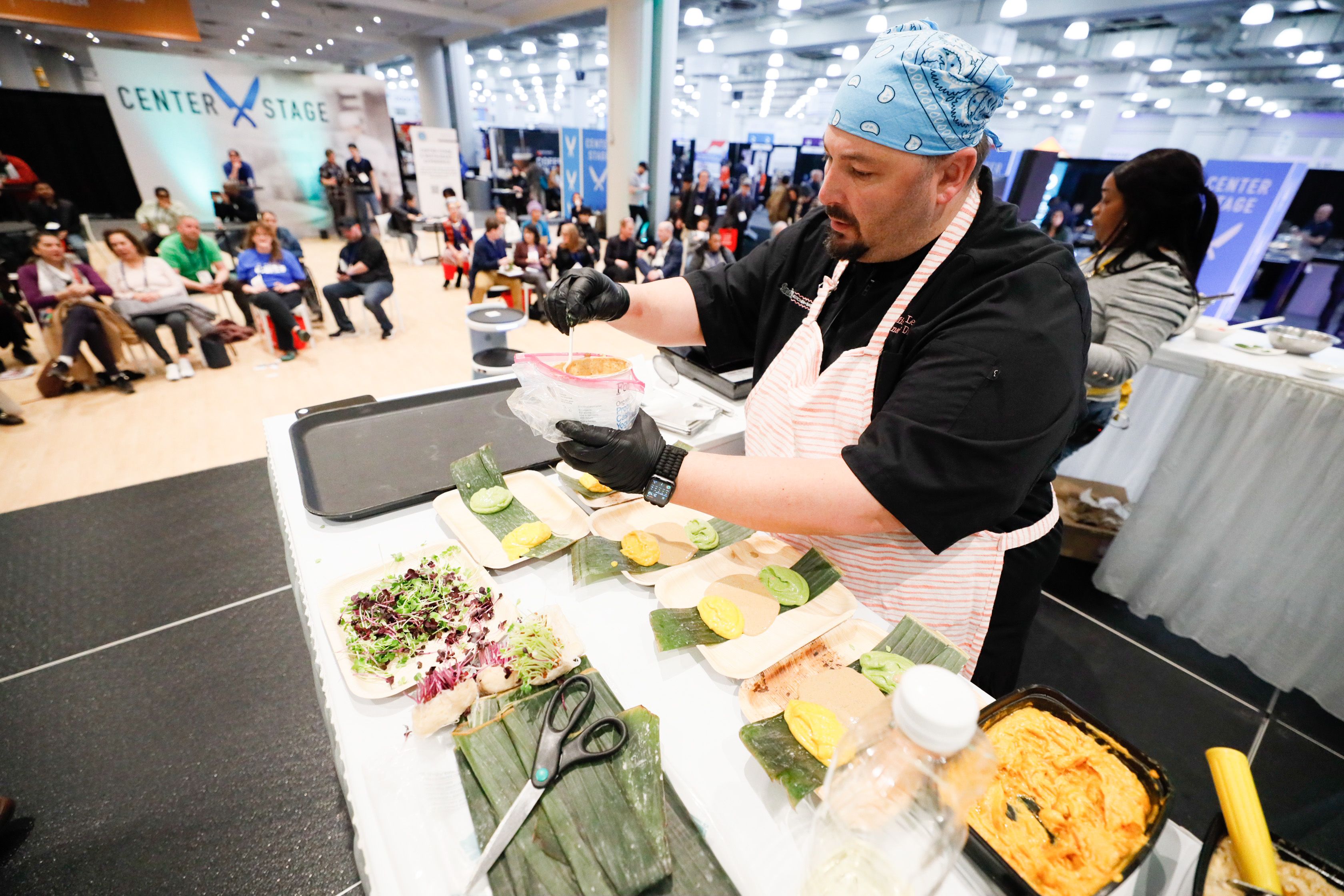The image captures a bustling scene at an exhibition hall called "Center Stage," featuring a culinary contest where chefs compete against each other. The spacious room is illuminated with numerous ceiling lights and prominently displays a large sign with the words "Center Stage" flanked by two crossed cooking knives. A significant audience, numbering around three dozen people, is seated in chairs, observing the event.

In focus is a close-up of a chef in the foreground, a white male wearing a blue bandana, black gloves, a black button-up shirt, a white apron, and an Apple Watch. His cooking station is cluttered with various utensils, including a pair of kitchen scissors and several trays with different foods. These foods include cabbages, some pastries, and green and yellow condiments. He appears to be handling something in a cup using either a fork or knife.

In the background stands another chef, a black female with long black hair, also engaging in the cooking competition. Both chefs are surrounded by an atmosphere charged with excitement and concentration as they showcase their culinary skills to the attentive crowd.